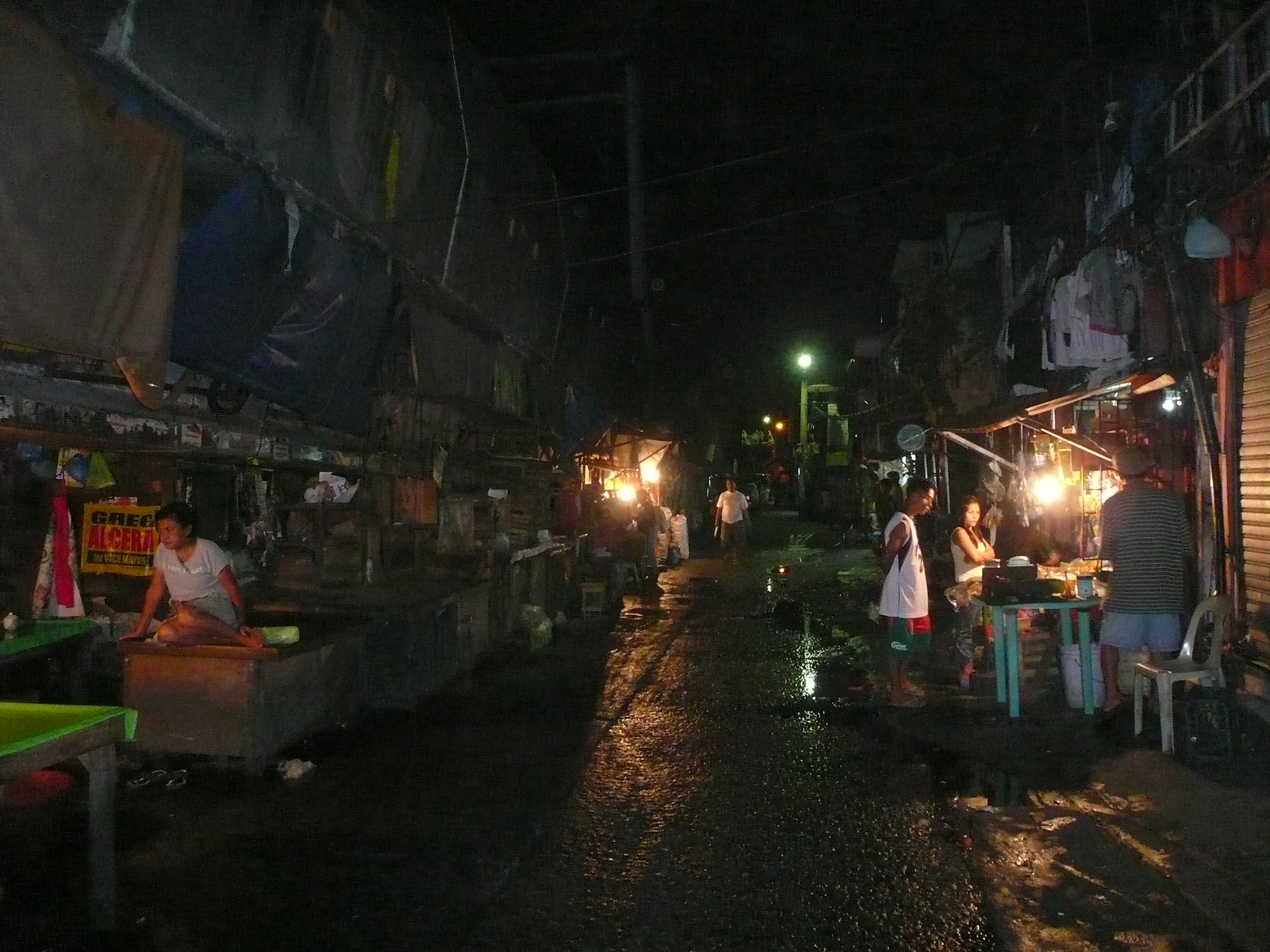This image portrays a bustling nighttime street, possibly situated in a Southeast Asian country like India. The scene is framed in a wide vertical rectangle, with a background of an inky black sky and a matching dark pavement that is dotted with water puddles. The street, lined with an economically modest atmosphere, features rows of street vendors on both sides, each with designated sections for their goods. Various tables display products, some illuminated by bright lights, while others remain dimly lit. On the left side, tan and blue tarps hang overhead, adding an eclectic touch to the setting. The right side of the street is notably marked by a metal awning sheltering a well-lit table, around which a group of three people stand, presumably examining items for purchase. Scattered throughout the scene are a few other individuals browsing the vendors' offerings, and distant street lights provide sporadic illumination, enhancing the nocturnal ambiance.